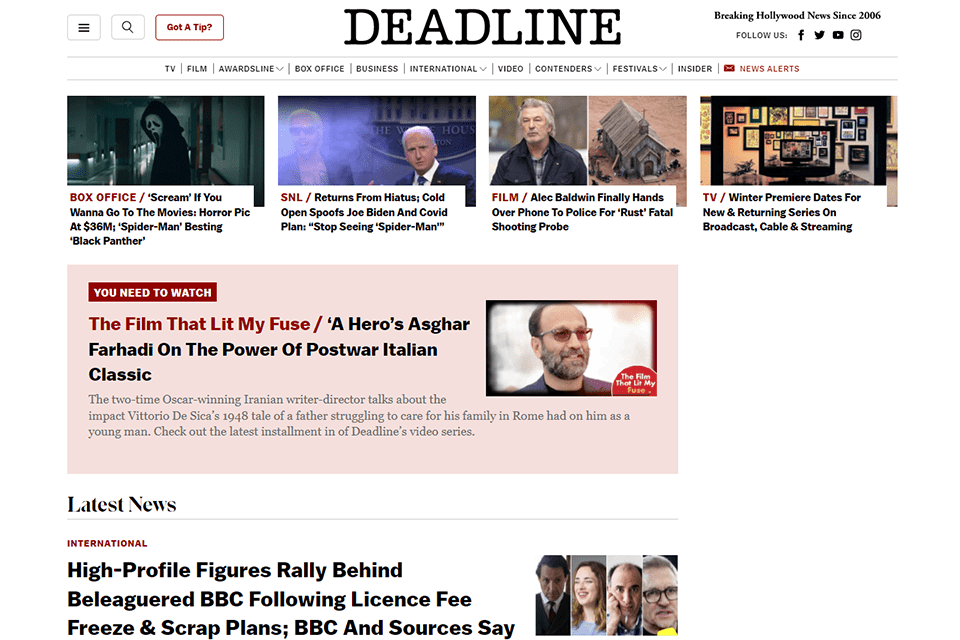This image captures a snapshot of a web page, likely from a news website, presented against a white background in a portrait orientation. The top section features a thin gray-bordered box, containing a hamburger menu next to a search icon. Adjacent to these icons is a red rectangular box with a white background and red text that reads "Got a Tip?". 

Central to the header is a black text title "Deadline," indicating the name of the website. Accompanying this title is the tagline "Breaking Hollywood News Since 2006," alongside icons for Facebook, Twitter, YouTube, and Instagram. Below the header, a thin gray line runs horizontally, segmenting the navigation bar, with clickable options including TV, Film, AwardsLine, Box Office, Business, International, Video, Contenders, Festivals, Insider, and News Alerts.

Beneath this navigation menu, thumbnail images link to various stories. The highlighted stories feature categories such as Box Office with a movie screen image, SNL, Film with a picture of Alec Baldwin, and TV. Below these story previews, a pink-highlighted box contains an article teaser with a red border at the top, titled "You Need to Watch." The article further expounds on a film reviving a post-war Italian classic and its potential to inspire. Lastly, the page includes a "Latest News" tab with further clickable content options, keeping readers engaged with current updates.